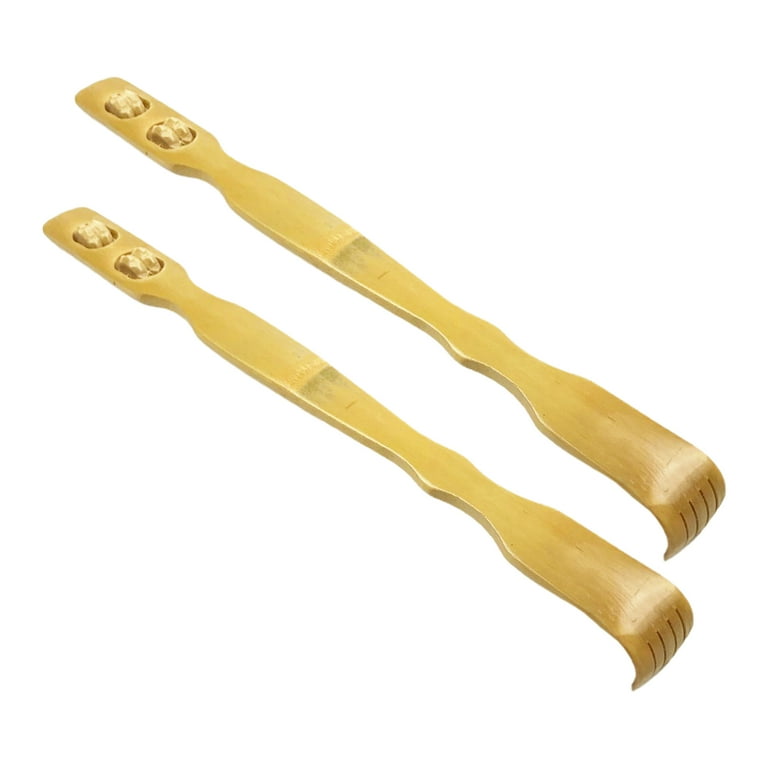This photograph showcases two intricately carved wooden back scratchers, displayed diagonally against a white background. Crafted from light-colored wood, possibly bamboo or pine, they are positioned with their handles pointing to the top left and the scratching parts aimed towards the bottom right. These back scratchers feature four distinct grooves at the scratching end, designed to provide effective relief. The handles are equipped with two wooden roller balls each, intended for massaging. The handles are slightly wider below the rollers and exhibit a gentle curvature, adding to their ergonomic design. The placement of the scratchers, one slightly ahead of the other, adds a dynamic visual element to the image.